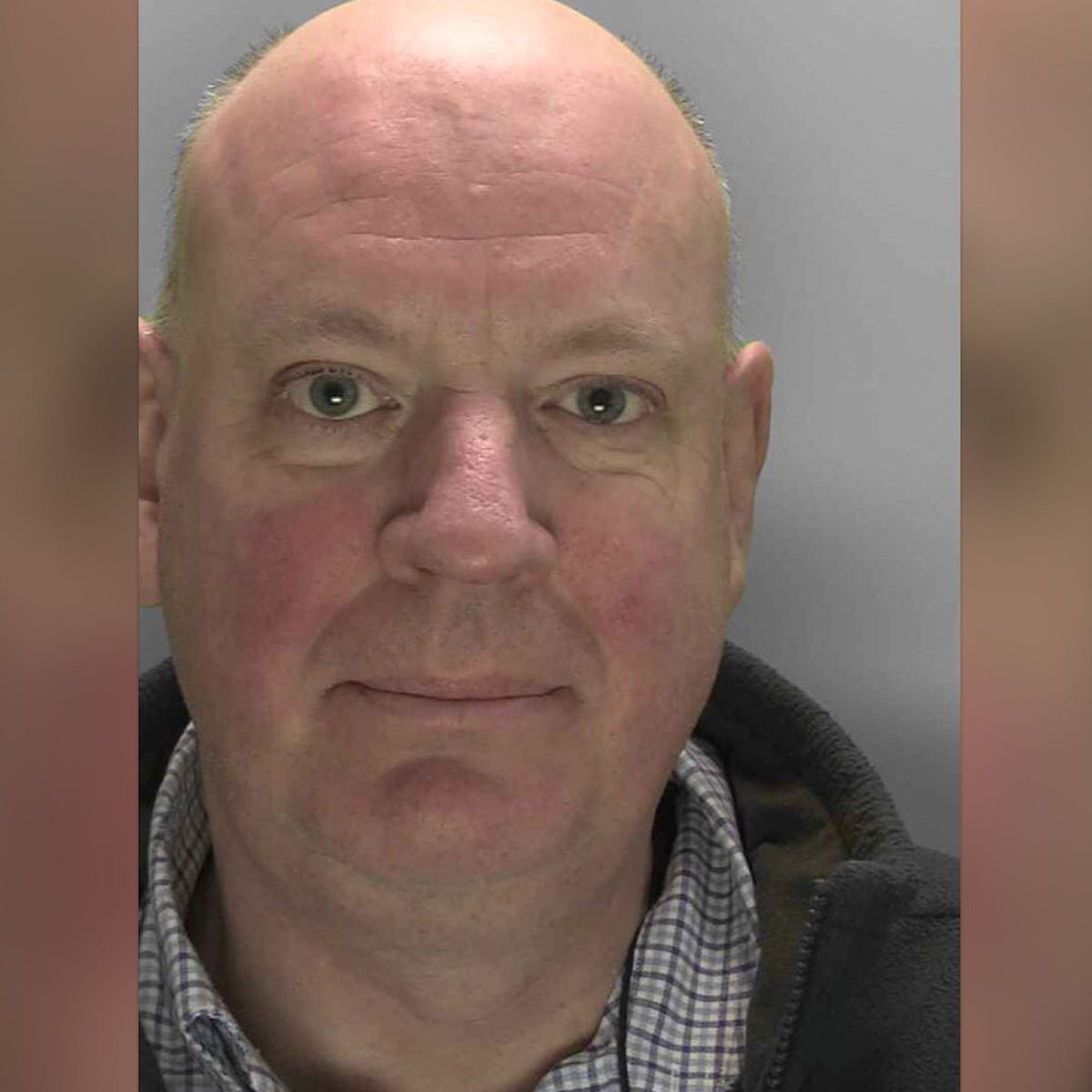The photograph showcases an older Caucasian male, likely in his late 50s or 60s, set against a neutral gray background. Positioned centrally in a close-up headshot, the man appears bald with a hint of stubble on the back of his head, characterized by salt and pepper hair. His complexion is somewhat ruddy and his face appears slightly puffy. He has light brownish-green eyes and very light eyebrows. His expression features a semi-smile with closed lips, directed intently at the camera. He is clean-shaven and dressed in a dark green fleece jacket with a zipper, over a checkered button-up shirt, which has a collar that is folded down and buttoned. The shirt features a pattern of green, light blue, and white checks, adding a bit of texture and color to his attire. The overall impression is that of a pleasant-looking gentleman engaging directly with the viewer.